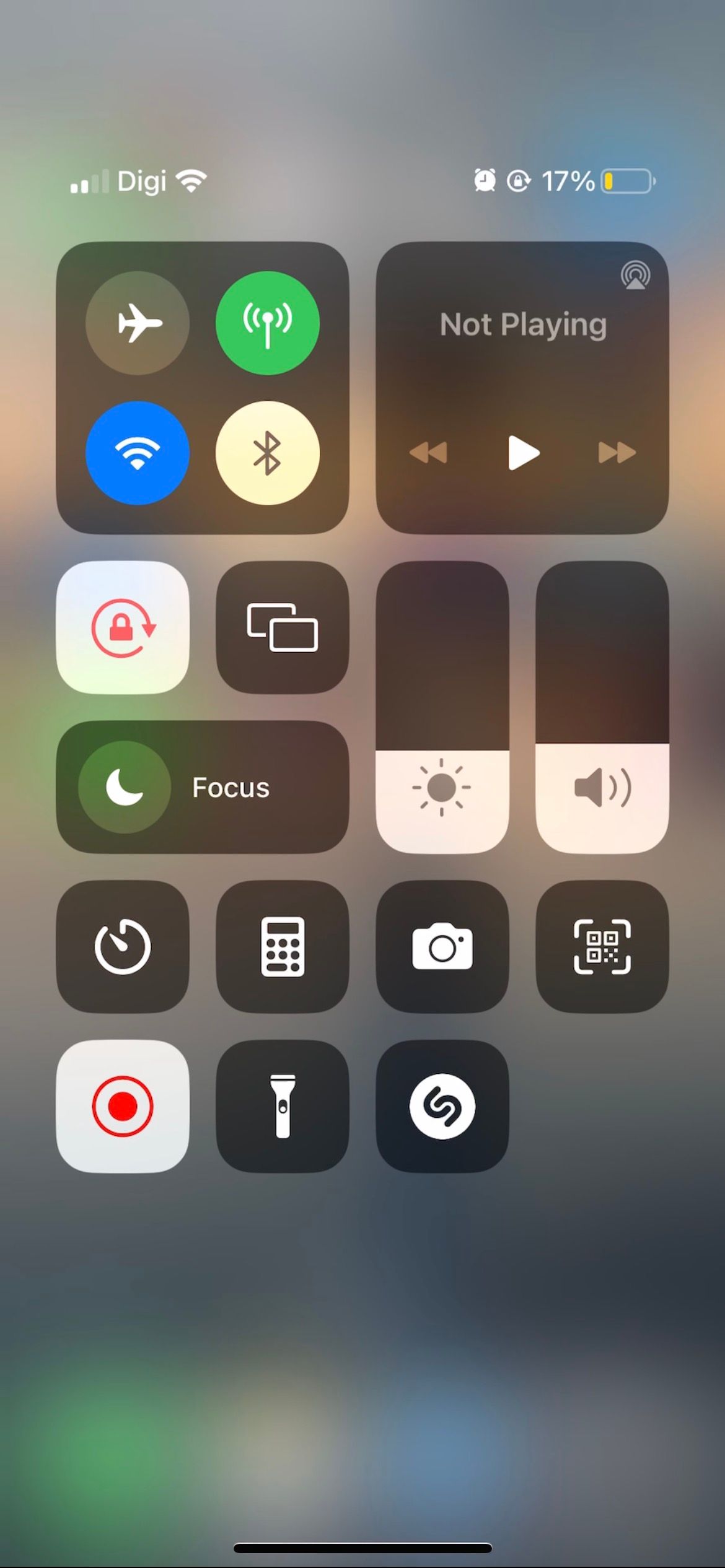The image depicts a smartphone screen displaying a segment of the settings page. Superimposed over a faint background of app icons and interface elements, the overlay appears somewhat translucent. At the top-left corner of the screen, the word "DIGI" is visible, accompanied by cellular signal bars and the Wi-Fi connectivity icon. Moving towards the top-right, the current time is displayed next to battery status indicators, showing a battery level at 17% with a yellow sliver indicating low charge.

In the central part of the screen, two rectangular sections divide various controls. The left section features four primary items: a green airplane mode icon, a green signal strength indicator, a blue Wi-Fi signal icon, and a Bluetooth icon. Alongside these, there are controls to adjust sound and screen brightness. Additional commonly used utility buttons are also present, including those for the flashlight, calculator, and camera.